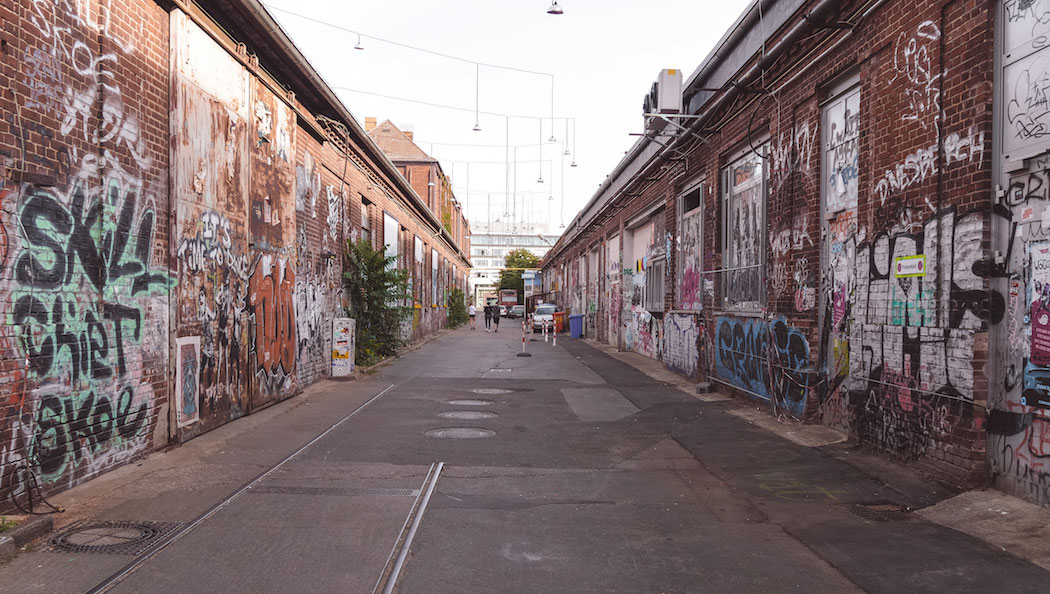The image captures a gritty alleyway scene from one end of the narrow passage. The ground is composed of classic dark gray concrete, while the walls on either side are made of brown bricks, each heavily adorned with various graffiti. One prominent piece of graffiti on the left wall reads "Skill Cheat Sko," rendered in black paint with a mint green border. The scene extends into the distance, where three small figures can be seen walking, scarcely distinguishable due to their distance. There is a parked car and some trash bins further down the alley, adding to the urban decay ambiance. Overhead, a couple of string lights stretch between the buildings, attempting to add a vestige of charm to the otherwise rundown area. The sky above is a bleak white-gray, contributing to the overall desolate feel of the scene. Despite some patches of green shrubbery sprouting from the cement, the presence of extensive graffiti and an unsettling atmosphere suggest this is not a particularly safe or welcoming area.